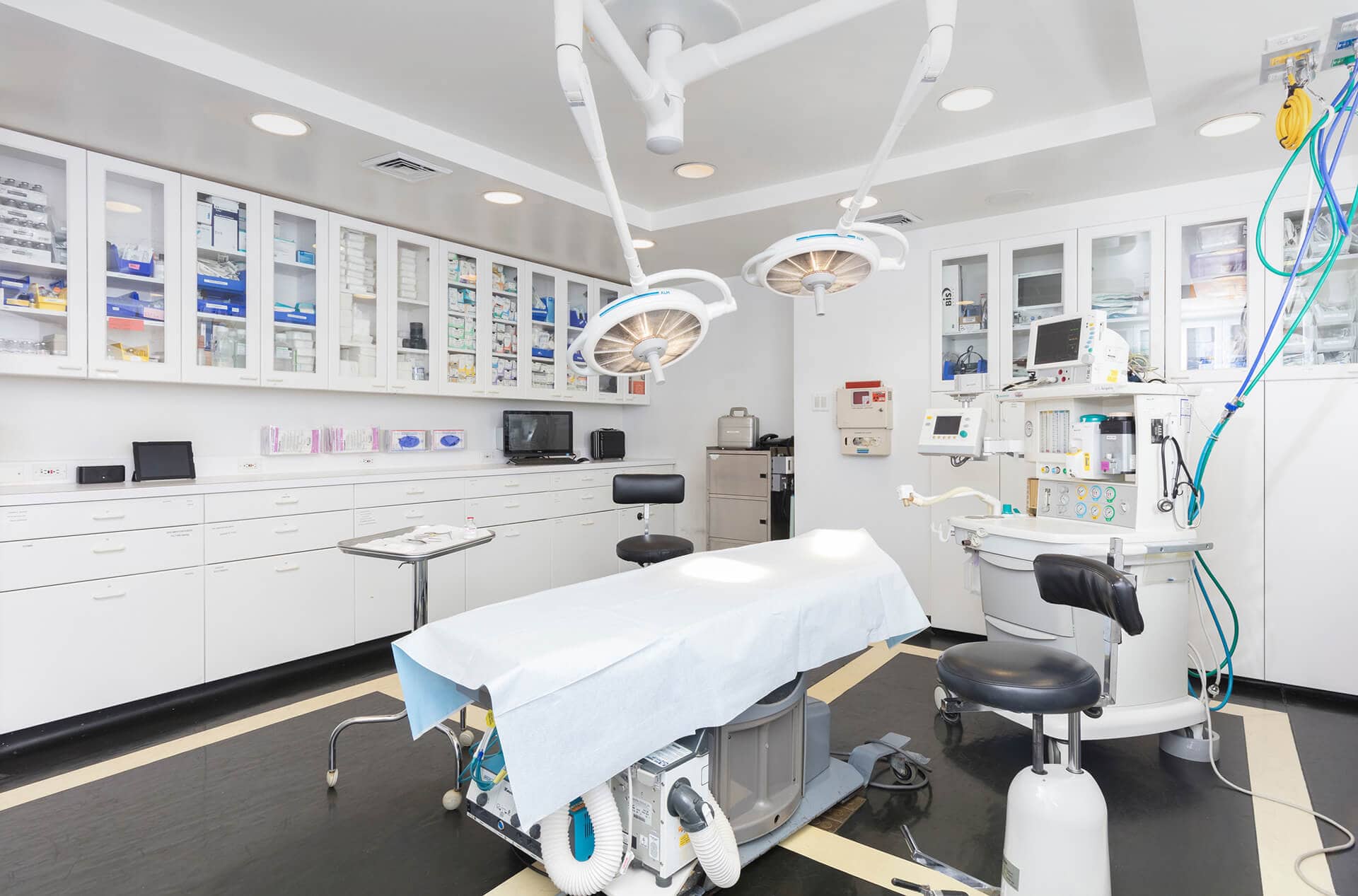The image depicts a modern medical examination or procedure room, likely from the last decade. Central to the room is a gurney covered with a white sheet, equipped with various medical devices including ventilation equipment and numerous wires, tubes, and buttons. Above the gurney, suspended from the ceiling, are two large, jointed, disc-shaped lights with an innovative design featuring illuminated fibers radiating from their centers, providing clear illumination for medical procedures.

To the left of the gurney is a compact metal tabletop supported by a unique, three-legged stand with wheels, presumably for easy mobility. A dark bluish-gray stool with a curved, partial backrest is positioned to the right of the bed, similar to another stool found behind the bed. Further back, there is a two-tiered workstation adorned with monitors, tubing, and medical apparatus.

The walls of the room form a corner on the right, each lined with vertically shaped windows near the ceiling, divided by white painted boards. These windows, potentially serving as cupboard doors, reveal multiple shelves stocked with various medical supplies, including numerous blue and a few orange boxes. Below the shelves, a continuous counter hosts additional equipment and paperwork.

The room features various other elements such as a black leather stool, a white plastic cabinet filled with medical supplies, and a small refrigerator topped with a light gray medical suitcase in the background. The ceiling is dotted with simple embedded lights, enhancing the overall illumination. The floor is primarily gray with a tan square around the workstation area, rounding out this well-equipped, sterile, and efficiently organized medical room.